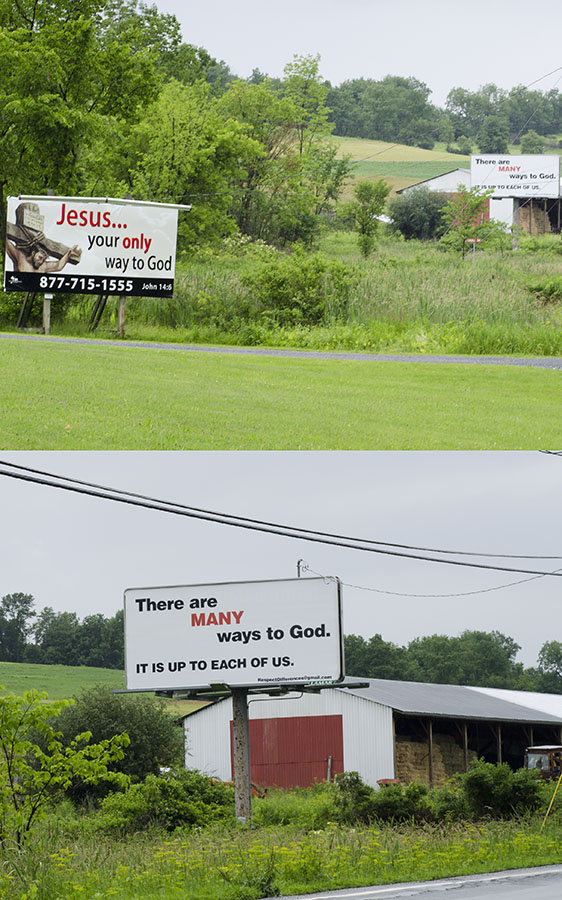The image consists of two photographs, arranged one above the other, each displaying billboards with pro-religion messages. 

In the top photograph, there are two distinct billboards seen from a distance. The nearest billboard, situated alongside a road, states, "Jesus, your only way to God," accompanied by a phone number and a biblical reference to John 14:6. The second billboard, positioned further away near a house, conveys a different message: "There are many ways to love God, it is up to each of us." Both billboards are placed along a street bordered by a verdant patch of greenery and scattered trees, contributing to a serene yet contrasting spiritual dialogue.

The bottom photograph is a close-up of the second billboard from the top image, offering a clearer view of the sign near the house. This closer perspective highlights the text promoting religious inclusivity against the backdrop of the domestic setting, underscoring the diversity of religious expression within the same vicinity.